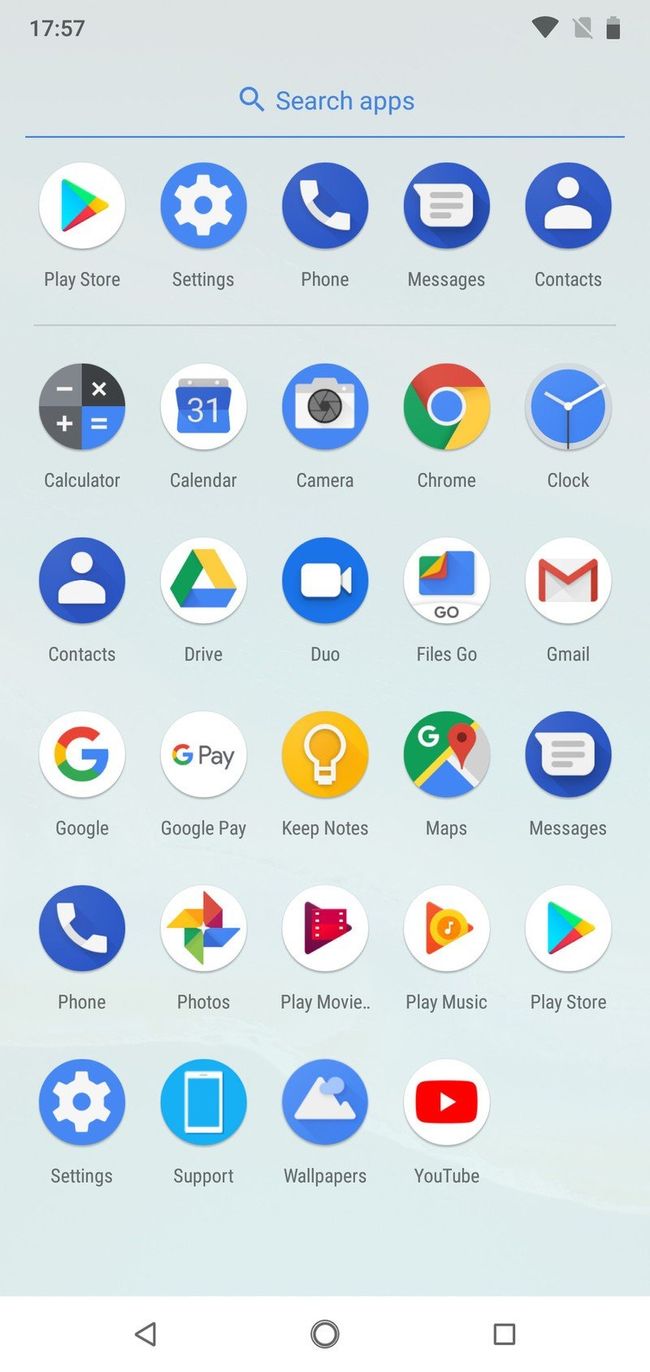This image displays the home screen of an Android device, potentially a Google phone. The screen is organized into a grid layout containing 29 app icons arranged in six rows. Each row contains five icons, except for the bottom row which has only four.

Starting from the top, the screen includes:
- **Top Row:** Play Store, Settings, Phone, Messages, Contacts
- **Second Row:** Calculator, Calendar, Camera, Clock, Files
- **Third Row:** Contacts, Drive, Duo, Files, Gmail
- **Fourth Row:** Google, Google Pay, Keep Notes, Maps, Messages
- **Fifth Row:** Phone, Photos, Play Movies, Play Music, Play Store
- **Bottom Row:** Settings, Support, Wallpapers, YouTube

Above the icons, there is a blue horizontal bar featuring a search field labeled "Search Apps," accompanied by a magnifying glass icon on the left for initiating searches.

The status bar at the very top of the screen shows the time as 17:57, a full Wi-Fi signal icon, a grey icon of an unknown function, and a battery icon indicating approximately 75% charge.

At the very bottom, there is a navigation bar with three icons: a triangle (back button), a circle (home button), and a square (overview button). The background of the screen is light blue, transitioning to slightly more vivid shades of blue towards the bottom.

The arrangement of the icons suggests they are likely sorted alphabetically.